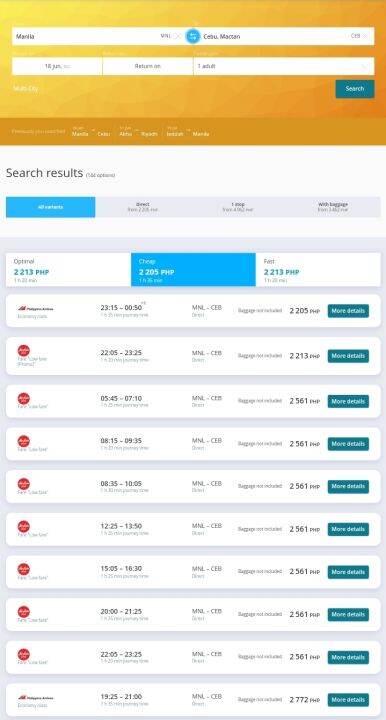This image appears to be a screenshot from a travel website. The top of the page features a yellow header containing white square boxes with text, which is not fully legible. Below this header is a blue search button with white text. Centered within the yellow header are six words, also unreadable.

Beneath the header, there's a section labeled "Search Results" with four interactive tabs. The first tab on the far left is highlighted in blue with white text. Below these tabs is a detailed table displaying various travel options, likely related to airlines. The table includes columns for start times, arrival times, departure and arrival destinations, and possibly airline codes.

Within the table, there's an option lit up in a blue background with white text labeled "Cheap," indicating it's the highlighted option. Each row in the table provides details about specific flights, including the airline name, start and arrival times, and the three-letter airport codes for departure and arrival locations. There are two additional columns, one displaying what seems to be a price, for example, "2205 PHP," suggesting the currency of the country. The final column offers a "More details" option for each listed flight.

Overall, the travel website offers a structured, user-friendly layout for comparing airline options based on various criteria such as cost, efficiency, and convenience.